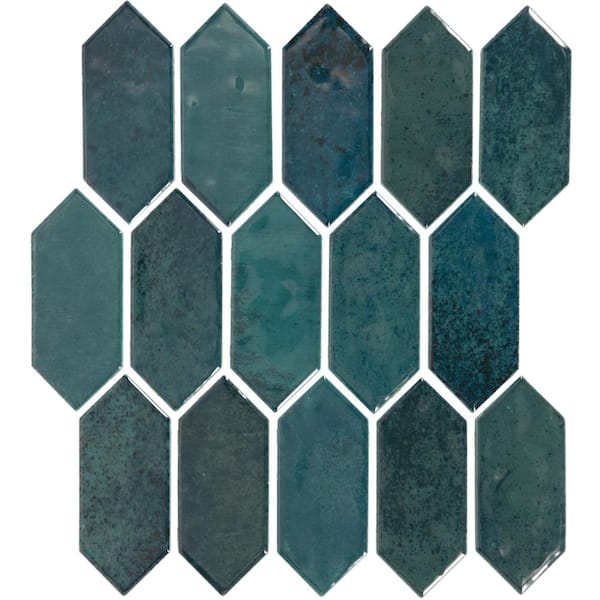The image features three rows of interlocking, elongated hexagonal tiles, each row containing five tiles. The overall arrangement forms a loose square without a definitive border, resting against a white background. These tiles are multicolored with a predominance of darkish, muted hues of blue, green, and brown. The texture varies slightly across the tiles, with random darker splashes creating subtle differences. The elongated hexagons are vertically stretched, resembling a marquee or diamond shape but not rounded. They nestle together precisely, creating a pattern where the tiles in the top row fit between those in the middle row, and this interlocking layout forms visible negative white lines between them. The color and subtle texture variations across the tiles add depth to the otherwise uniform pattern, making it suitable for an accent wall.